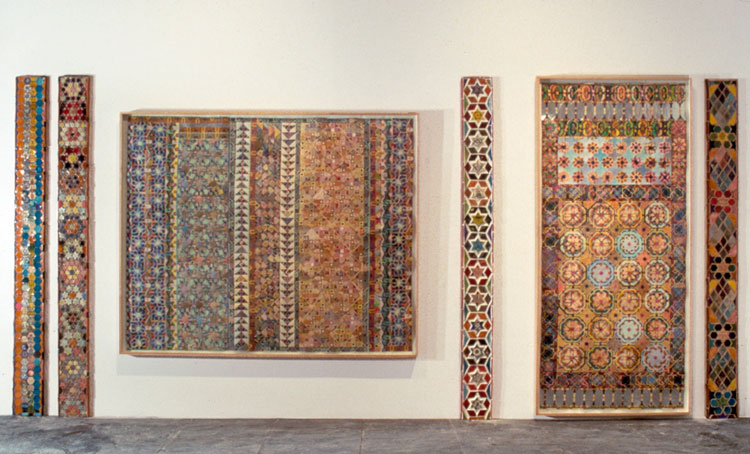This image is a color photograph of a textile installation titled "Whitney Biennial Installation" by Joyce Kozloff, created in 1979. Displayed in a museum-like setting, the installation features a series of intricately designed textiles against a beige wall. The artwork includes multiple elongated rectangular pieces, primarily in a vertical orientation with vibrant multicolored patterns. 

From left to right, the pieces showcase various intricate designs and motifs:
- The two vertical strips on the left exhibit rich patterns in brick red, aqua, and a multitude of other colors, almost floral and geometric in nature.
- A central large horizontal panel presents a tapestry with vertical stripes in blues and beiges, segmented into multiple narrow sections with detailed, varied designs.
- Adjacent to this is another vertical piece with a beige background adorned with multicolored symbolic imagery.
- Further right, a tall strip features stars within pentagon shapes against a vibrant, multihued backdrop.
- The final piece on the right is a long vertical installation on a black background with motifs in gold, red, and blue, resembling flowery and emblematic designs.

The textiles exhibit a rich tapestry of design elements and colors such as turquoise, orange, yellow, red, maroon, and grays. This installation exemplifies the pattern and decoration style, creating a visually captivating display of modern textile art.